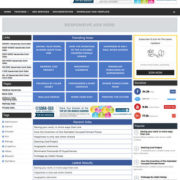The image presented is of a highly blurred and low-quality page, primarily dominated by a white background interspersed with multiple colors. Central to the image are approximately 12 blue boxes, each containing white text, although the specific wording is illegible. Above this cluster of blue boxes is a long horizontal gray box extending from the left to the right edge of the image, with a smaller black box positioned directly above it spanning the same width. To the left of the central blue boxes, there are three additional black boxes, each accompanied by black text beneath them. On the right side of the blue boxes, a yellow outlined box frames a certain area, emphasizing its contents. Below this yellow box, several colored circles—blue, light blue, orange, and red—are visible in a row. Despite the overall blurry quality obscuring precise details and text, the arrangement of colors and boxes makes the structure of the page partially discernible.